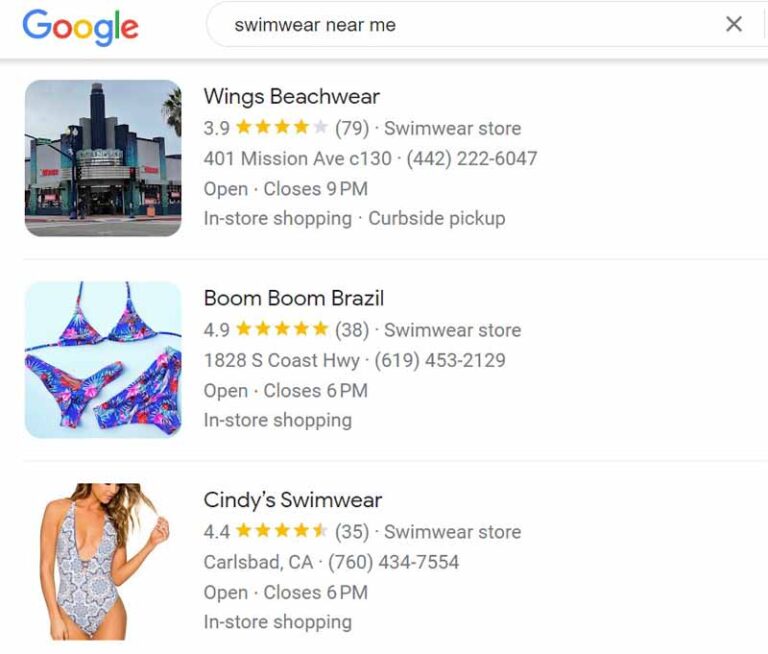A detailed screen capture of a Google search query for "swimwear near me." The image is roughly square-shaped with a white background, featuring black and gray text. In the upper left corner, the Google logo is visible, with each letter in a different color—blue, red, yellow, blue, green, and red. To the right of the logo, the search bar displays the text "swimwear near me." 

Below the search bar, three search results are presented, each accompanied by a square-shaped thumbnail on the left. The first result shows an image of a storefront located on a city street corner. This search result is for "Wings Beachwear." 

The second result features a picture of a multi-piece bathing suit, comprising a bikini top and two bottoms in a floral blue and pink print. This entry pertains to "Boom Boom Brazil." 

The third image displays a model— a white woman with long, dark blonde hair—wearing a one-piece swimsuit in light gray and blue with a low-cut V-neck. This result refers to "Cindy's Swimwear." 

Each store result includes a black header with the store's name, followed by a yellow star rating and smaller gray text detailing the store's information.